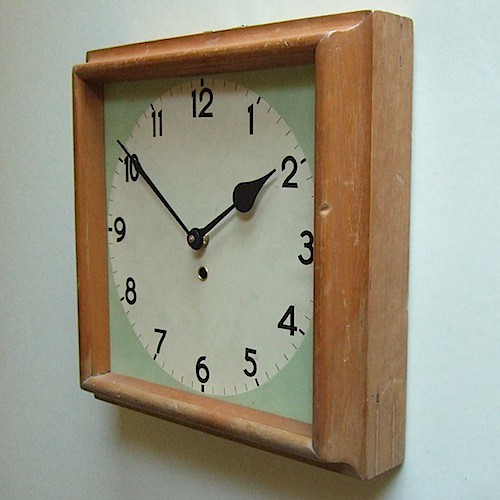A slightly skewed angle photograph captures a small wall clock with a thick, weathered wooden frame. The clock face is bordered by a light green rim, adding a touch of color contrast to the white background. Black numerals and clock hands stand prominently against the white face, ensuring easy readability. The image is well-lit, suggesting it was taken indoors, possibly near a window where natural light enhances the scene. The photograph is of moderate quality, clearly highlighting the intricate details and textures of the clock's frame.